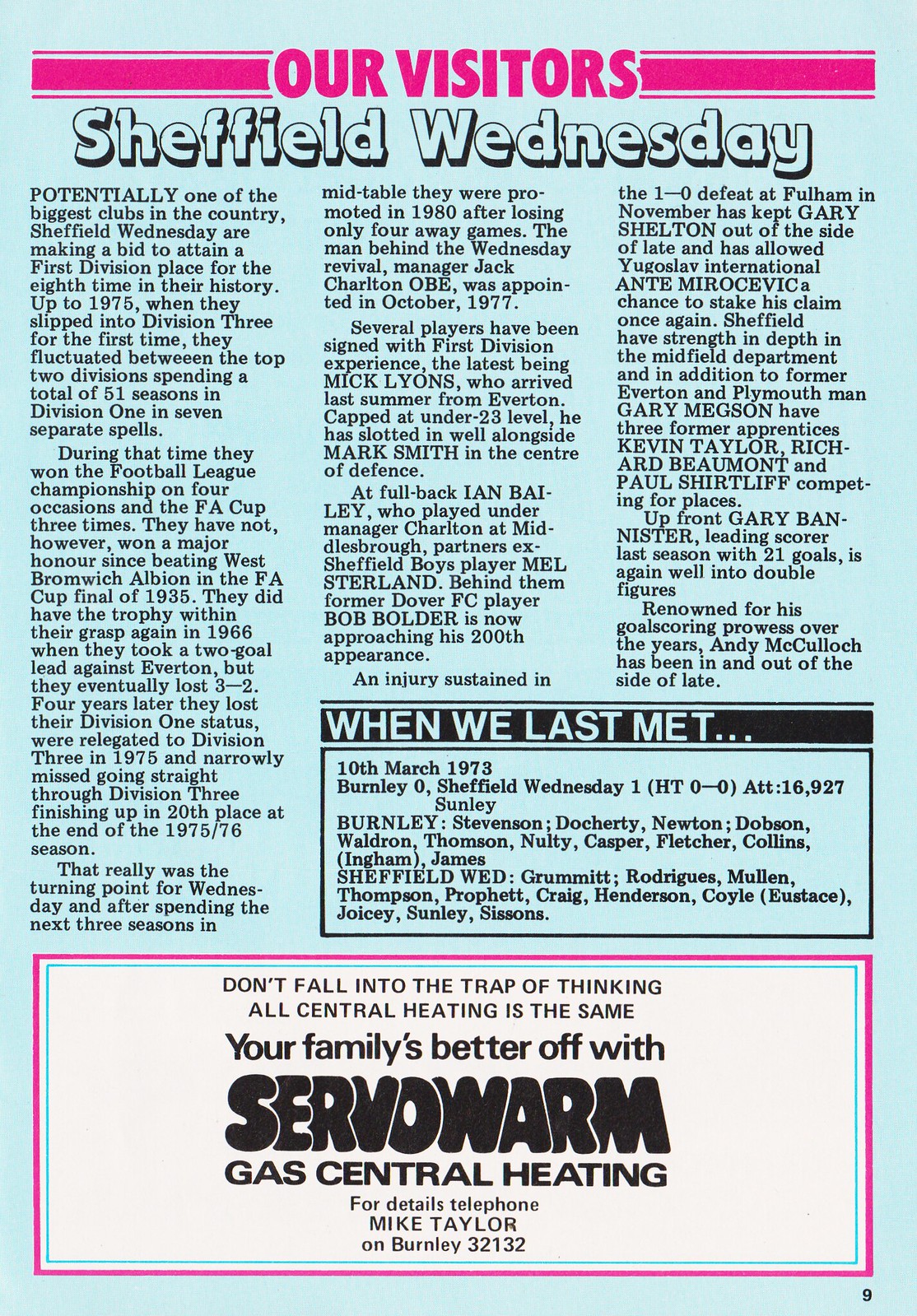This is a nostalgic scan of page nine from an old magazine or program, characterized by its predominantly blue background and vibrant pink text header that reads "Our Visitors." Centered below this, in eye-catching outline text with a drop shadow, it announces "Sheffield Wednesday." The page features an engaging article detailing Sheffield Wednesday, touted as "potentially one of the biggest clubs in the country," as the football club endeavors to secure a First Division spot for the eighth time. This informative piece continues over several paragraphs. Further down, in a bordered section titled "When we last met," the page recalls a match dated 10th March 1973, where Burnley and Sheffield Wednesday ended the first half in a zero to zero draw, ultimately concluding with Sheffield Wednesday's 1-0 victory. A white box at the page's bottom presents an advertisement, urging readers with the slogan, "Don't fall into the trap of thinking all central heating is the same. Your family's better off with Servo Warm gas central heating," and includes contact information for the company.